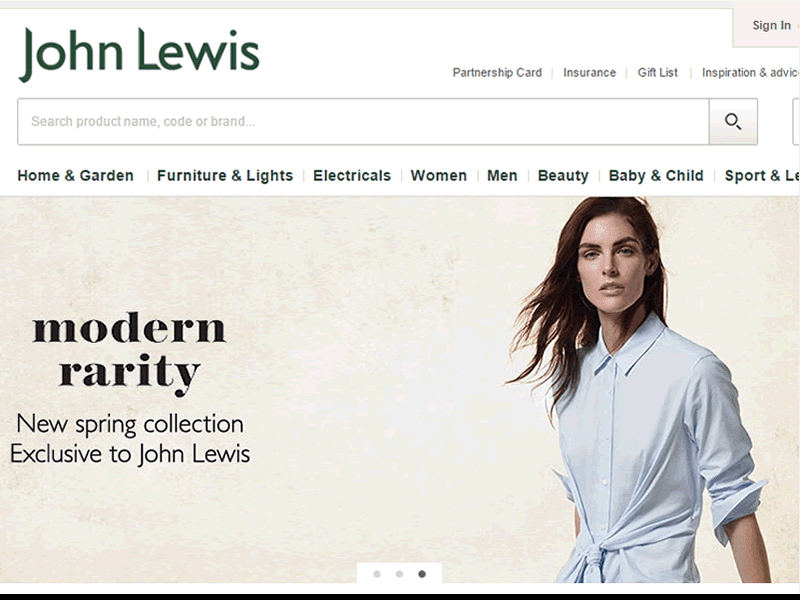This screenshot from a website features the John Lewis header prominently. At the top, a white rectangle spans the width of the page. In the upper left corner, "John Lewis" is written in large black font. To the right of the brand name are several clickable links: "Partnership Card," "Insurance," "Gift List," "Inspiration," and "Advice." In the upper right corner, there is a "Sign In" option.

Beneath the John Lewis logo, there is a search field encased in a black rectangle with gray text that reads, "Search product name, code, or brand." A magnifying glass icon is positioned at the right end of this field.

Following the search bar, there is a site map featuring clickable categories: "Home and Garden," "Furniture and Light," "Electrical," "Women," "Men," "Beauty," "Baby and Child," "Sports," and another partially visible category starting with "LE."

Below the site map, an advertisement displays a striking image of a white woman with flowing black hair, appearing to be in her mid-twenties. She gazes directly ahead while wearing a cinched, one-piece button-up dress resembling a man's office shirt that transitions into a dress at the bottom. The text to the left of her reads, "Modern Rarity, New Spring Collection, Exclusive to John Lewis."